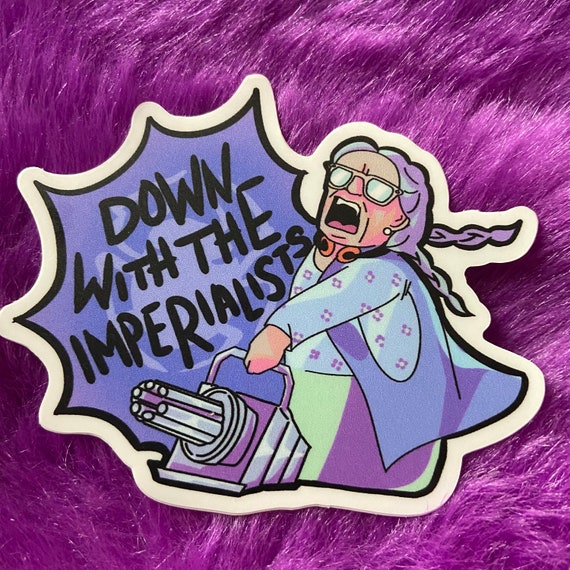The image is a close-up photograph of a sticker lying on bright purple, textured fur that resembles a wig or a shag rug. The sticker itself features a detailed, cartoonish depiction of an elderly woman with long white hair in braided pigtails, wearing tan-rimmed glasses and a single pearl earring. Her mouth is wide open as if she is shouting, with the black text "Down with the imperialists" displayed to the left of her. The woman is dressed in a light blue shirt with pink dots, a blue vest, and a green skirt, and she's wielding a silver and purple minigun. The sticker has a blue background, a black and white border, and an irregular starburst shape with peaks and valleys around the edges. The overall scene is vibrant, with the bright purple fur accentuating the colors of the sticker.